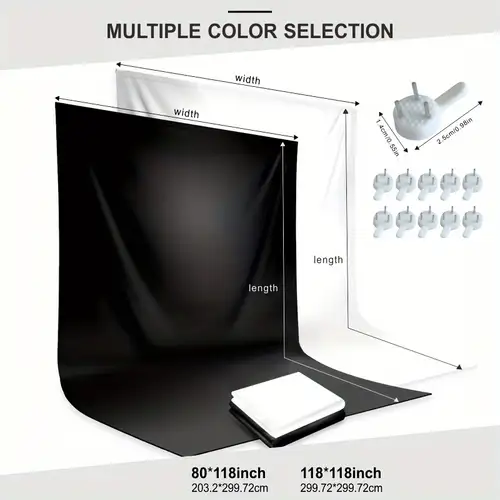This detailed image appears to be an advertisement for photography backdrops, prominently featuring a top caption that reads "Multiple Color Selection." The ad showcases two backdrop options: a larger white cloth measuring 118 inches by 118 inches or 299.72 by 299.72 centimeters, and a smaller black cloth measuring 80 inches by 118 inches or 203.2 by 299.72 centimeters. These backdrops are designed to hang and curve under, creating a seamless background for objects placed on them. The image also displays accessories to the right, depicting ten round, white brackets with three prongs on top and a protruding piece on the side. These brackets are detailed in an enlarged photo and measure 1.4 centimeters by 2.5 centimeters or 0.55 inches by 0.98 inches. Additionally, a laptop is seen positioned on the black backdrop, emphasizing practical use. The overall layout suggests that the ad is targeting professional photographers looking to equip their studio with versatile and durable backdrops.